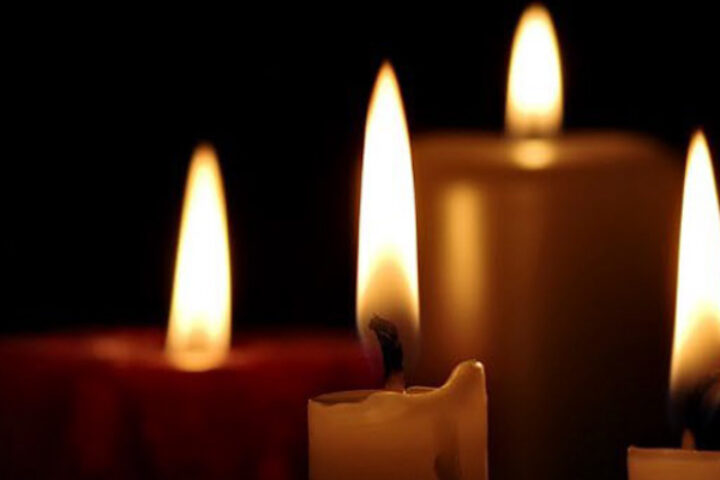This is an up-close, professional photograph of four lit pillar candles against a black backdrop, arranged horizontally. The foremost candle is a narrow, slightly melted ivory pillar with a jagged top, displaying a high, orange flame atop its lit wick. Positioned to its immediate left is another ivory candle, already burned lower, with a similarly high, orange flame. In the blurred background on the right, a wide, red pillar candle with a low white flame stands out. To the left, a thick, tall cylindrical orange candle with a shorter flame completes the scene. The detailed interplay of flames highlights the colors varying from white-hot to orange-red, capturing the intricate, captivating essence of burning candles.